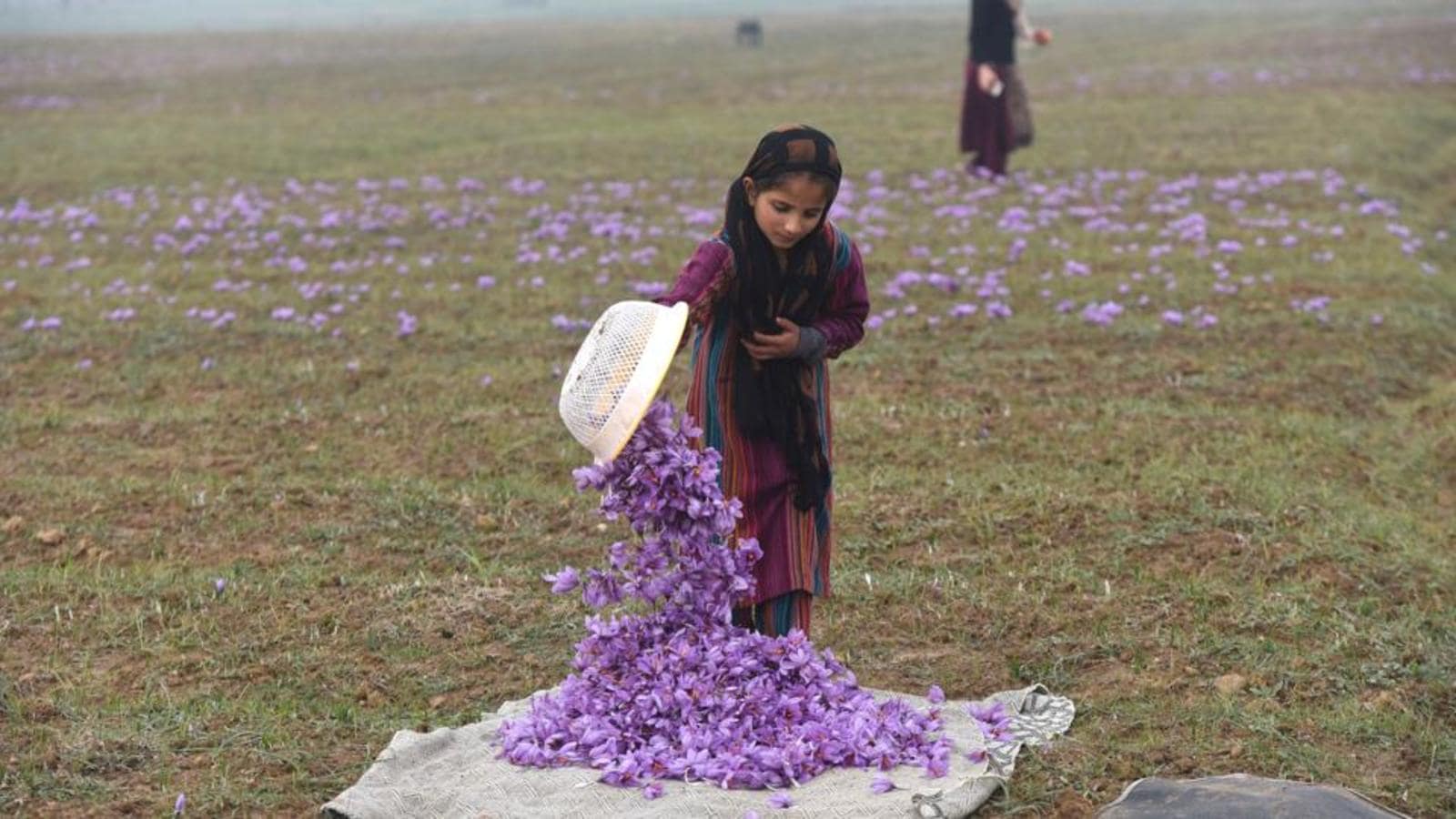In the photograph, a young girl with long dark brown hair, dressed in a maroon robe accented with teal, kneels on a grassy field scattered with purple wildflowers. She is pouring a basketful of these vibrant lavender flowers onto a white cloth, possibly a blanket or animal skins, displaying a dynamic sense of movement as the flowers cascade from the white plastic basket. Surrounding her in the background is a field organized with sections of purple flowers, and we can also see an adult figure, likely her mother, partly visible and similarly dressed. The adult woman appears to be collecting flowers as well, adding to the serene yet industrious scene of harvesting flowers, possibly for sale or decorative use. The idyllic setting emphasizes the beautiful flow and coordination in their activity amidst the stunning natural backdrop.